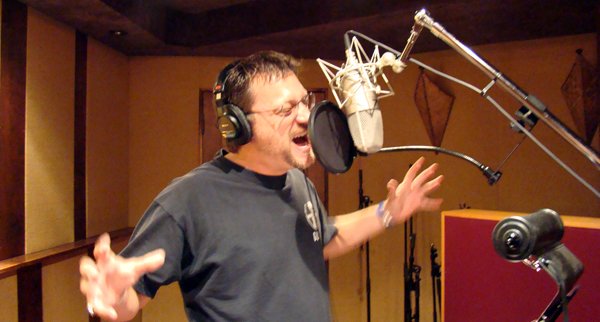In this detailed image, a man is captured singing passionately in a professional recording studio. He stands alone, eyes closed, with glasses on and his mouth wide open, revealing his upper and lower teeth. He sports short, slightly spiky brown hair, held with some gel, and wears a gray t-shirt with a logo on the right side, along with a blue wristband and a watch. The man has headphones on and is positioned in front of a sizable silver microphone equipped with a black pop filter. In front of him are likely lyrics he's reading from and a red stereo amp. The background features soundproofed brown and tan walls, ensuring no external noise disrupts the recording. The photograph is horizontally oriented, capturing this intense moment of musical expression in great detail.